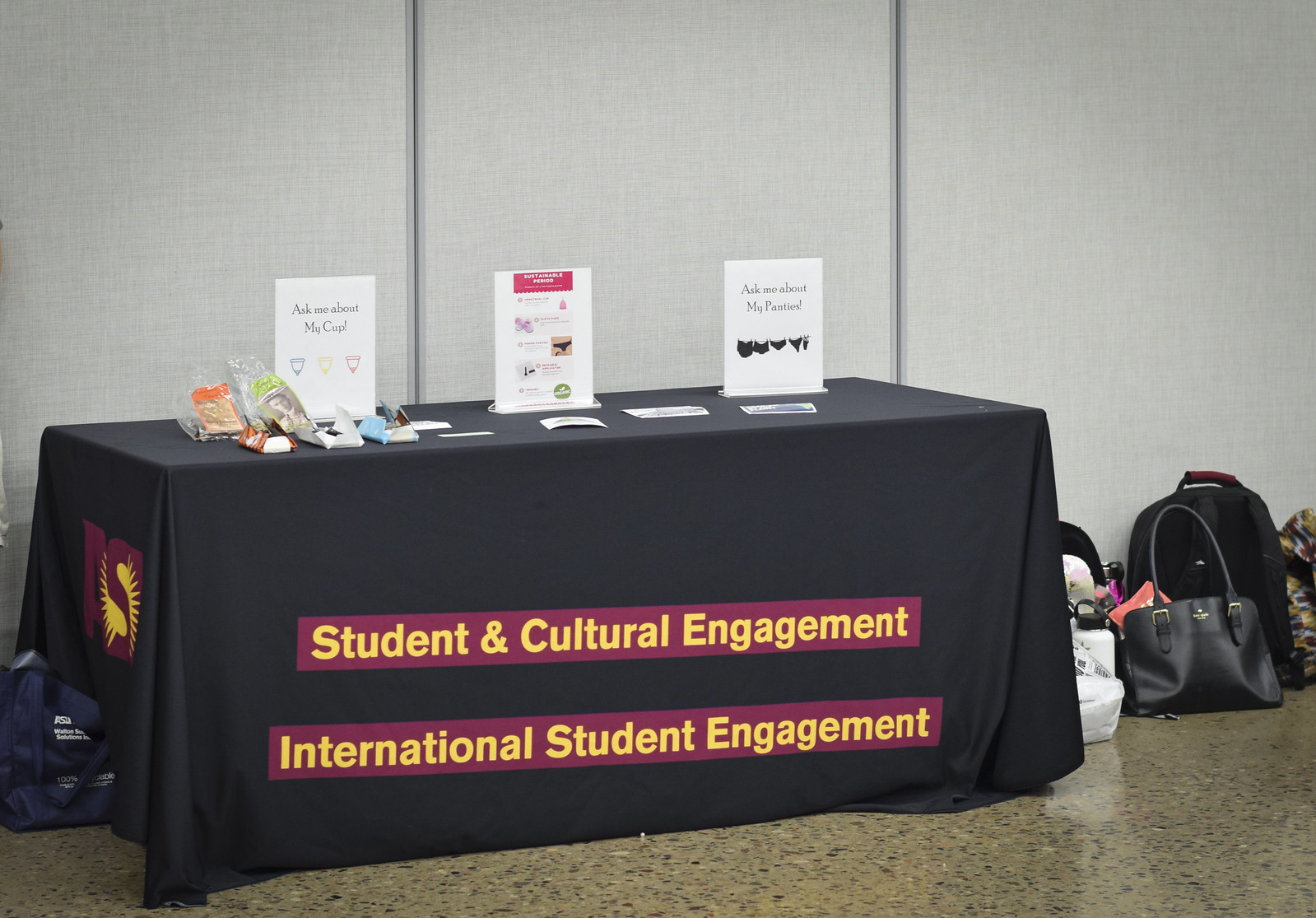The image depicts a display table at an event, likely on a college campus, covered with a black cloth. The banner draped over the front of the table is emblazoned with the words "Student and Cultural Engagement" and "International Student Engagement" in red and yellow text. On the table, three upright signs encased in plastic are prominently featured. The first sign reads "Ask Me About My Cup," accompanied by images of blue, yellow, and red menstrual cups with the caption "Sustainable Period." The second sign says "Ask Me About My Panties," and features a clothesline displaying various types of underpants. Scattered across the table are some papers and open plastic bags, and nearby lies a collection of personal items including two backpacks, a purse, and two water bottles, one white and one pink. To the right of the table, several bags are also visible on the floor, possibly belonging to the individuals managing the display.